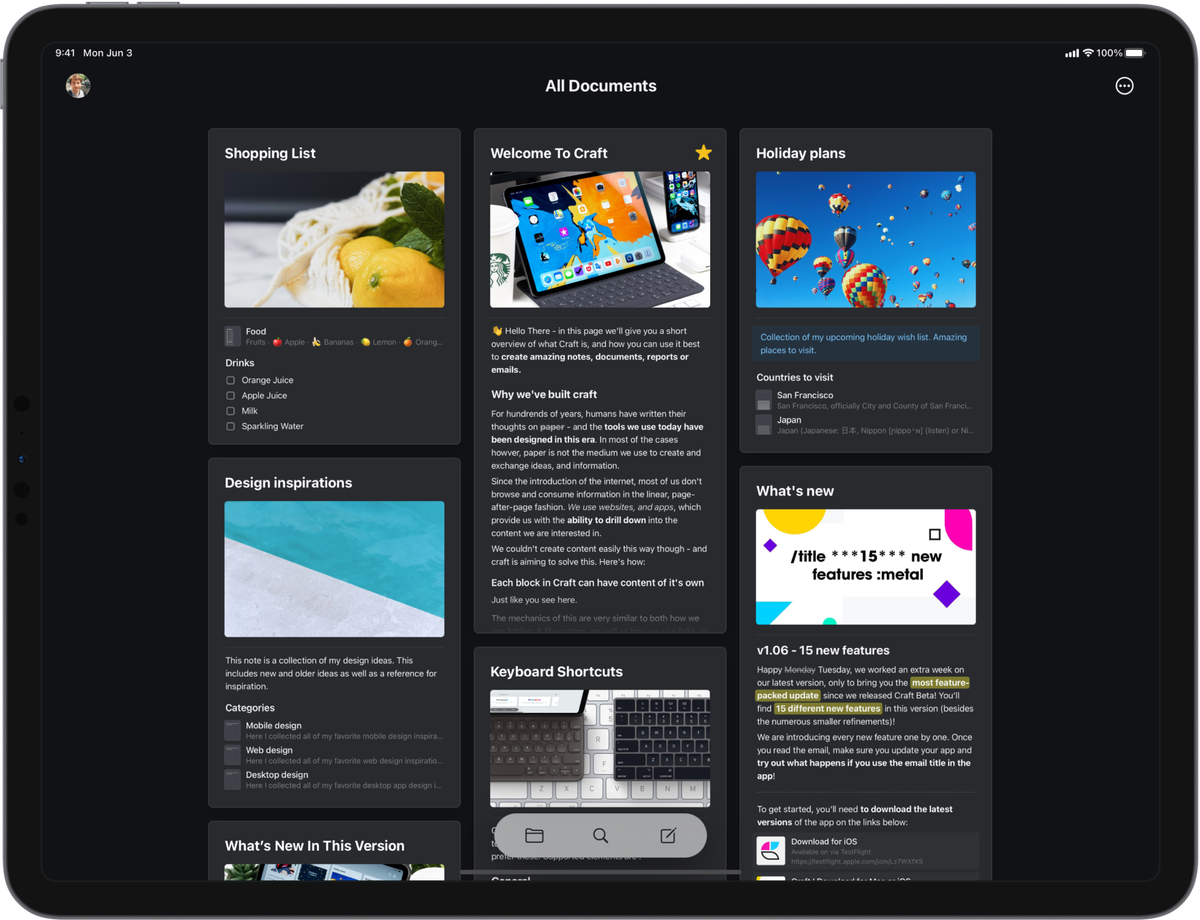A detailed webpage is displayed on the screen, featuring multiple sections and thumbnail images. In the top-left corner, a horizontal black bar contains essential information, including "941 MON June 3rd" in white font at the top-right. To the left of this date and time, icons for a power button, and volume control buttons are visible. Further to the right, signal strength is indicated by four bars, and a battery icon to its right shows 100% charge in gray.

Beneath this section, a thumbnail depicts lemons inside a fabric bag. At the top-left of this thumbnail, the heading "Shopping Lists" appears. Below the image, the category "Food" is followed by several gray icons with corresponding labels: an apple and the word "apple," a banana and "banana," a lemon and "lemon," and an orange and "orange." Further down, under a section titled "Drinks," a list is displayed with four empty checkboxes beside items: "Orange Juice," "Apple Juice," "Milk," and "Sparkling Water."

Moving down the page, the title "Design Inspirations" introduces the next thumbnail, showcasing the side of a pool. In gray text, a note reads: "This is a collection of my design ideas. This includes new and older ideas as well as references for inspiration." Below this, a section titled "Categories" in white has three empty checkboxes next to headings: "Mobile Design," "Web Design," and "Desktop Design."

In the middle of the page, a title "All Documents" in white precedes another thumbnail labeled "Welcome to Craft," featuring images of a cell phone and tablet. Accompanying text in gray reads: "Hello there. In this page, we'll give you a short overview of what Craft is and how you can use it best to create amazing notes, documents, reports, or emails. While we've built Craft, for hundreds of years, humans have written their thoughts on paper, and the tools we use today have been designed in this era. In most cases, however, paper is not the medium we use to create and exchange ideas and information. Since the introduction of the internet, most of us don't browse and consume information in the linear, page-after-page fashion. We use websites and apps, which provide us with the ability to drill down into the content we are interested in. We couldn't create content easily this way, though, and Craft is aiming to solve this. Here's how."

Bold white text below declares: "Each block in Craft can have content of its own." Following this, gray text reads: "Just like you saw here." The remaining portion is cut off.

Further down, another thumbnail titled "Keyboard Shortcuts" appears, illustrating a keyboard and various icons (file, search, and edit). To the right, a thumbnail labeled "Holiday Plans" shows hot air balloons, with blue text below stating: "Collection of my upcoming holiday wish list, amazing places to visit." In white, the heading "Countries to Visit" precedes two empty checkboxes labeled "San Francisco" and "Japan." Smaller text below is too small to decipher.

At the bottom-right, a final thumbnail titled "What's New" appears. It features a picture with a white background, yellow half-moon, white square, purple diamonds, and other shapes. Text inside the image reads: "/title ***15*** new features; metal." Below, in white, it continues: "V1.06215 new features," followed by partially readable text: "Happy..." (the rest is too small to read). An explanation in gray reads: "Tuesday, we worked an extra week on our latest version, only to bring you the most feature-packed update since we released Craft. Here's..." (the remaining part is too blurry to make out). The update mentions "15 different new features" highlighted in green, along with numerous smaller refinements, encouraging users to update the app and explore the new features.